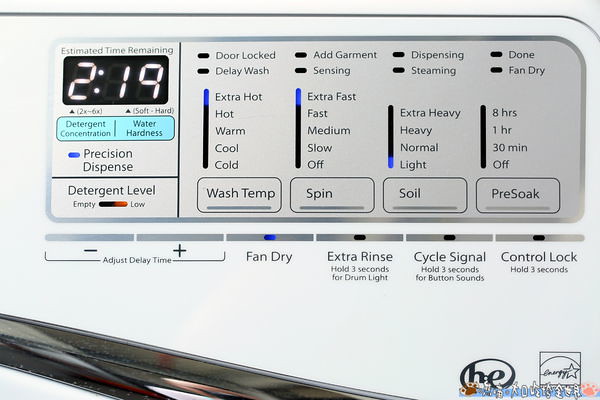The image displays a comprehensive advertisement for a high-efficiency, ENERGY STAR-rated washing machine. Dominating the center is a digital timer displaying "219" minutes, with "Estimated Time Remaining" written above in black letters on a white background. To the left, in a blue oval, are options for "Detergent Concentration" and "Water Hardness." Right below that, "Precision Dispense" is highlighted with a blue light next to it, and "Detergent Level" is marked with a red light indicating "Low." Prominent labels and lights span across the machine's interface, indicating various settings and statuses such as "Door Locked," "Delay Wash," "Add Garments," "Sensing," "Dispense," "Streaming," "Done," and "Fan Dry." 

On the washer's setting panel, options to adjust washing parameters include "Wash Temp," ranging from "Extra Hot" to "Cold," and "Spin Speed," from "Extra Fast" to "Off." Soil levels can be set from "Extra Heavy" to "Light," and "Pre-Soak" times range from "8 Hours" to "Off." Additional features like "Extra Rinse," "Drum Light" (hold for 3 seconds), "Cycle Signal," "Button Sounds," and "Control Lock" (hold for 3 seconds) are also included. The display incorporates English and Chinese characters, emphasizing the machine's international usability. The Energy Star logo at the bottom right corner highlights its energy efficiency.